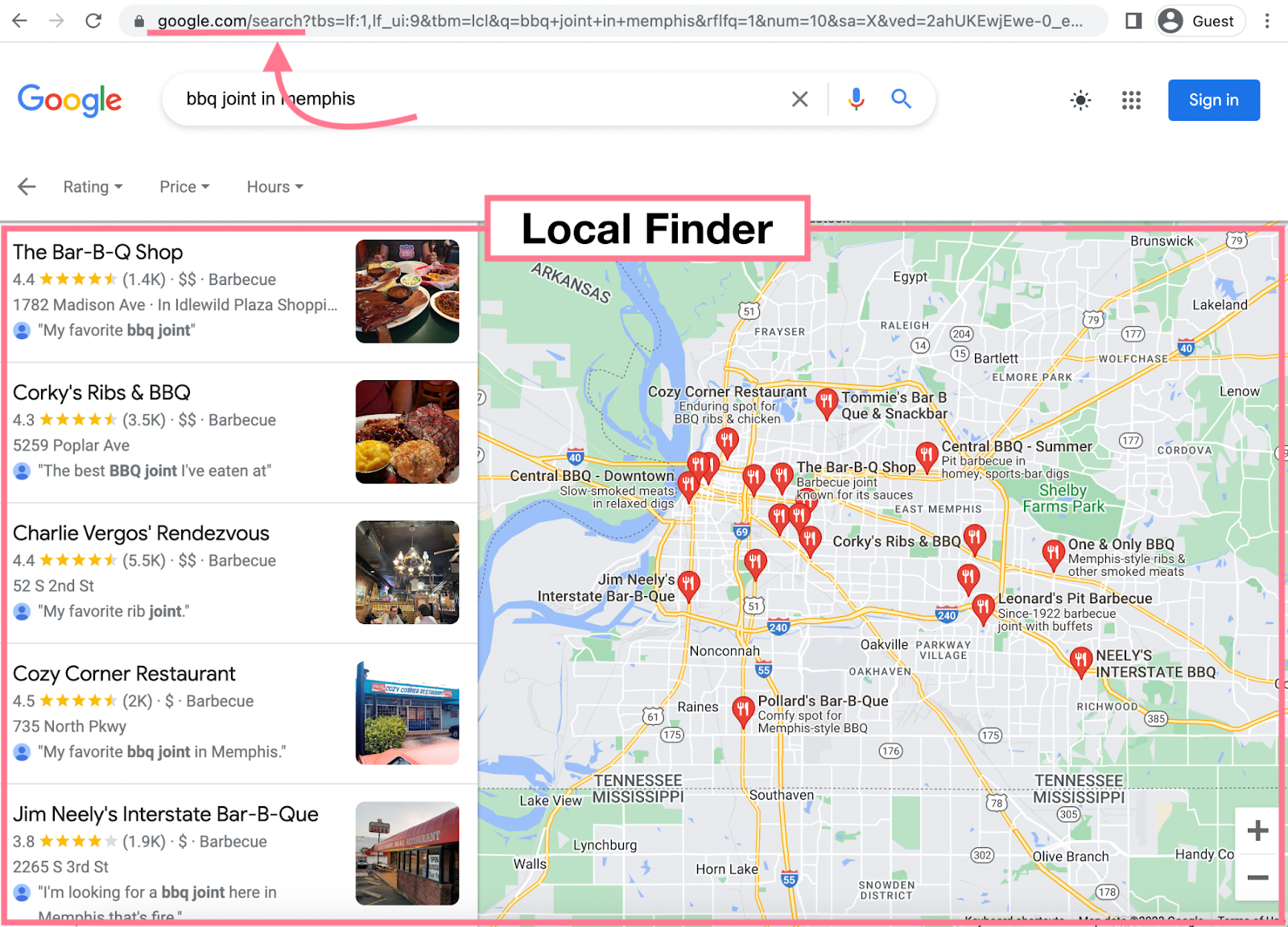This is a detailed screenshot from Google Maps on a web browser, showcasing several key elements on the screen. At the top, you can see the browser's toolbar featuring a back arrow, a forward arrow, and a refresh button. Next to these icons, there is the address bar displaying the following URL: "google.com/search?tbs=lf:1,if_ui:9&tbm=lc&q=bbq joint in memphis&rlfq=18&um=10&sa=X&ved=2ahUKEWE_jewE-0...". On the upper right corner of the toolbar, there is a silhouette of a person with the label "Guest" beside it.

Below the toolbar, the Google logo is prominently displayed, accompanied by a search field where the query "barbecue joint in Memphis" is entered. Additionally, there is a small, green, Photoshopped arrow pointing upwards, highlighting the "google.com/search" URL in the address bar.